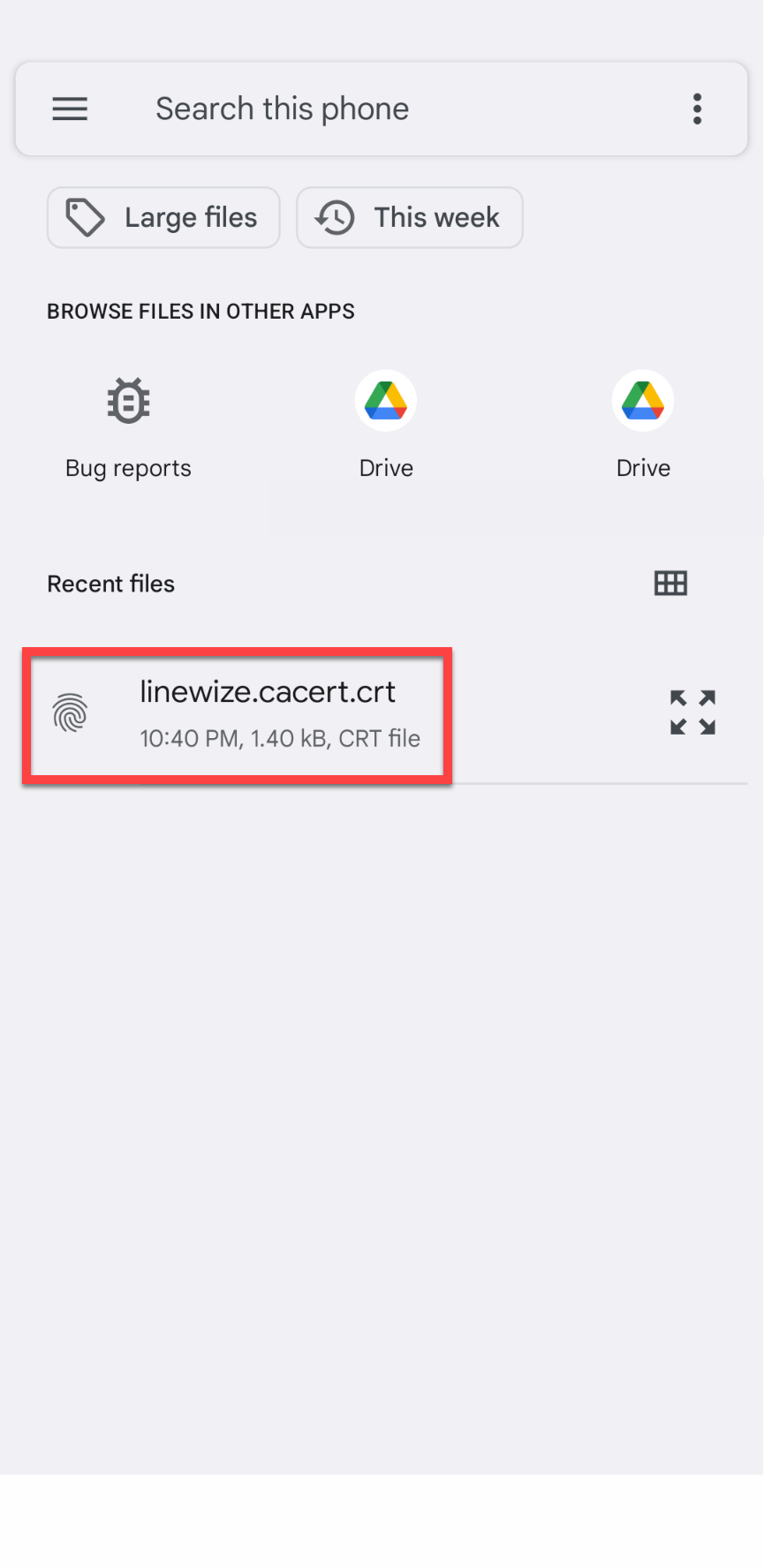The image features a gray background with several user interface elements arranged in a structured manner. At the very top, there is a search bar, resembling a window with three horizontal black lines on the left side. This bar contains the text "Search this phone" in black lettering, and on the right side, there are three thick black lines indicating additional menu options.

Beneath the search bar, there is a section with two gray-outlined boxes. The first box is labeled "Large files," and the second box, similar in appearance, is labeled "This week." Below these boxes, in bold black lettering, are the words "Browse files and other apps."

Following this section, the screen presents a labeled area titled "Bug reports" which includes an icon of a bug. Next to this is the label "Drive" accompanied by a colorful triangle icon in shades of red, yellow, and green, symbolizing the Google Drive logo. The same "Drive" label with its logo is repeated above this section.

Further down, there is a box with a red outline. Inside this box is the text "mine wise concert crt 10 40 p.m 140 kilobytes." Adjacent to this, on the right side, there is a segmented area with six smaller slots, though the specifics within these slots are not detailed. The rest of the image maintains a uniform gray background.